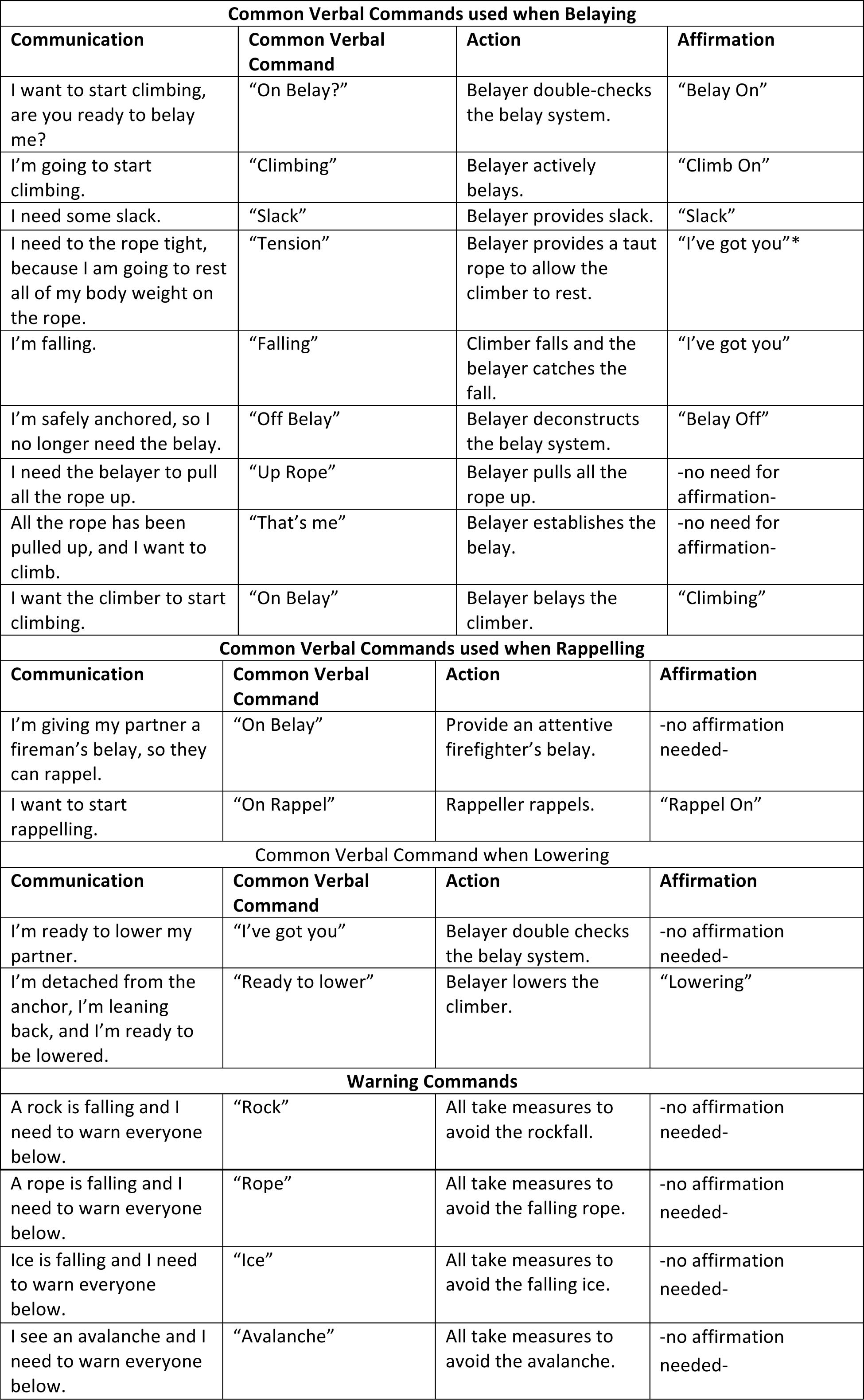This black and white image showcases a detailed chart titled "Common Verbal Commands Used When Playing," segmented into four main sections: "Common Verbal Commands When Belaying," "Common Verbal Commands When Repelling," "Common Verbal Commands When Lowering," and "Warning Commands." Each section is further divided into four columns: "Communication," "Common Verbal Command," "Action," and "Affirmation." 

The "Belaying" section, which is the most comprehensive with approximately nine rows, begins with "I want to start climbing. Are you ready to belay me?" under Communication. The corresponding verbal command is "On belay," the action is "Belayer double checks the belay system," and the affirmation, in quotes, is "Belay on."

The "Repelling" section includes commands like "I'm giving my partner a fireman's belay so they can repel." Here, "On belay" serves as the verbal command, while the action is "Provide an attentive firefighter's belay," and no affirmation is required.

In the "Lowering" section, a command example is "I'm ready to lower my partner." The verbal command is "I've got you," with the action being "Belayer double checks the belay system," and again, no affirmation is needed.

Finally, the "Warning Commands" section covers actions such as "A rock is falling and I need to warn everyone below," where the verbal command "Rock" is followed by the action "Take measures to avoid the rock fall," without requiring an affirmation.

This detailed chart appears to be a crucial reference for individuals working in the rock climbing industry, ensuring effective and standardized communication during various climbing activities.